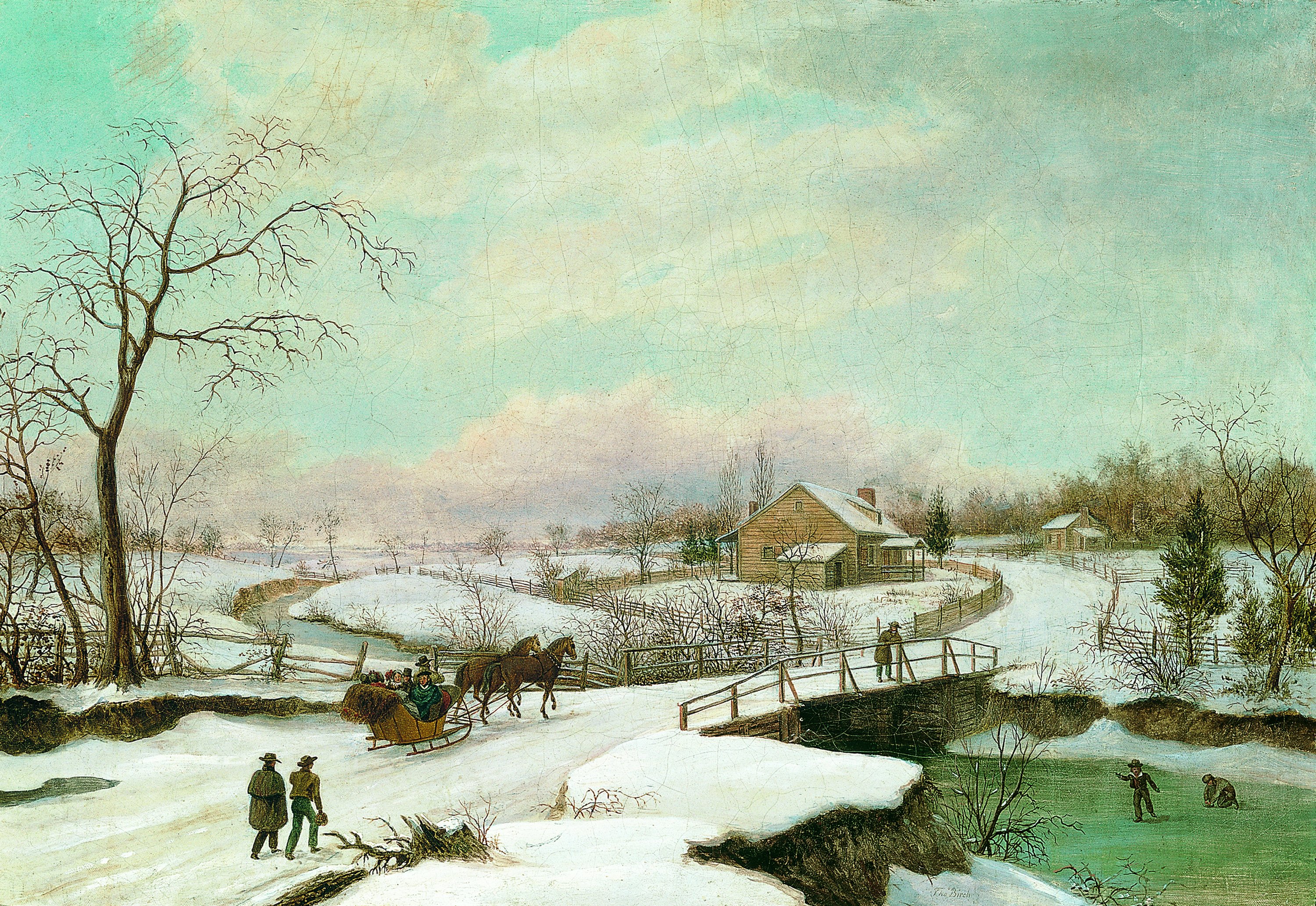This captivating painting depicts a serene country winter scene characterized by a snow-covered landscape under a sky transitioning with shades of pink, blue, and gray. Central to the image is a yellow or beige farmhouse with a brick chimney, surrounded by a few outbuildings. The snowy ground is dotted with bare trees, though a few retain green leaves. A wooden bridge with railings spans a small creek that runs through the scene, adding a nostalgic touch.

In the foreground, two horses are pulling a brown, open sleigh carrying about six people. Nearby, a couple of children are playfully ice skating on the frozen creek, while others are walking towards the farmhouse. One person stands on the small wooden bridge, taking in the peaceful surroundings. The sky, filled with white clouds, hints at a recent snowfall, creating an enchanting, picturesque country landscape.